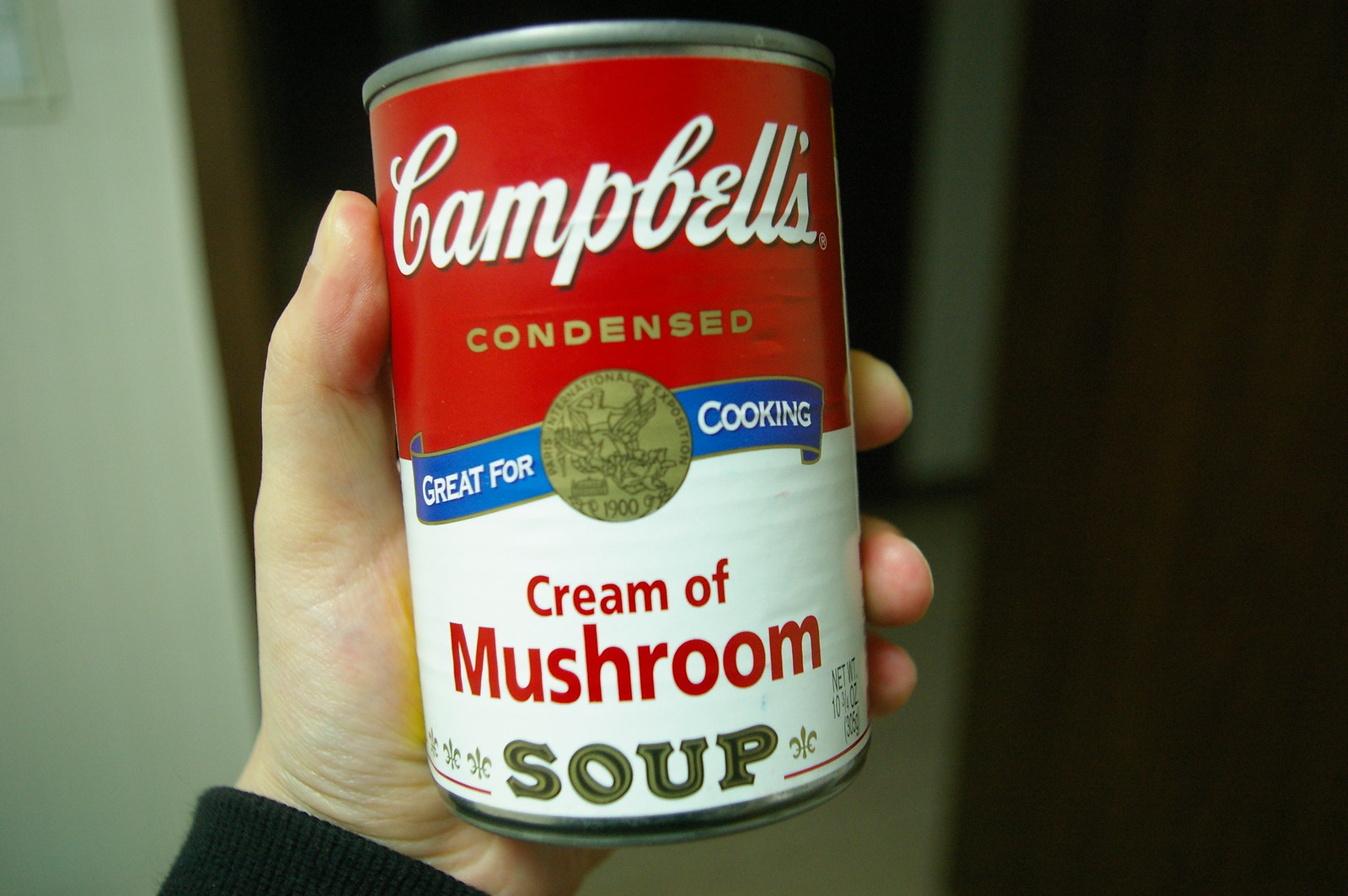In this photograph, a hand is prominently holding an aluminum can of Campbell's Cream of Mushroom soup. The can captures the eye with its iconic design: the top portion is wrapped in a bold red background, featuring the word "Campbell's" elegantly scripted in white cursive letters. Directly beneath that, the word "Condensed" is highlighted in gold lettering. A small blue banner further accentuates the can, bearing the phrase "Great for Cooking" and a central gold emblem. The lower half of the can is white with the words "Cream of Mushroom" emblazoned in red, juxtaposed above "Soup," which is written in a striking combination of gold and black. The hand holding the can shows the details of the fingers and a part of the wrist, which is dressed in a black long-sleeved shirt. The background of the image is softly blurred, suggesting the interior of a home with subtle hints of a wall and doorway visible in the out-of-focus areas.